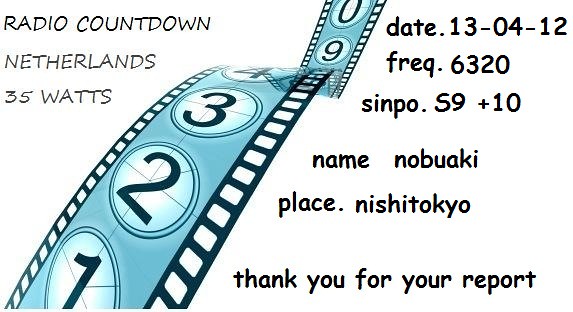The image appears to be a hybrid of a meme or advertisement, heavily text-based, featuring a prominently illustrated film strip running diagonally from the top center to the bottom left. The film strip is colored in shades of blue and white, with numbered circles ranging from 1 to 9, cycling back to 0, resembling an old-school film reel. 

In the top left corner, there is black text on a white background stating, "RADIO COUNTDOWN, NETHERLANDS, 35 WATTS." Meanwhile, on the right side of the image, additional information is presented in black Comic Sans font: the date "13-04-12," frequency "6320," and "S-I-N-P-O: S9 plus 10." The name "Nobuaki," the place "Nishitokyo," and the message "Thank you for your report" are also included, all in the same Comic Sans font.

The intricacies of the illustration together with the detailed text create a unique and engaging visual, blending retro film aesthetics with precise technical information.